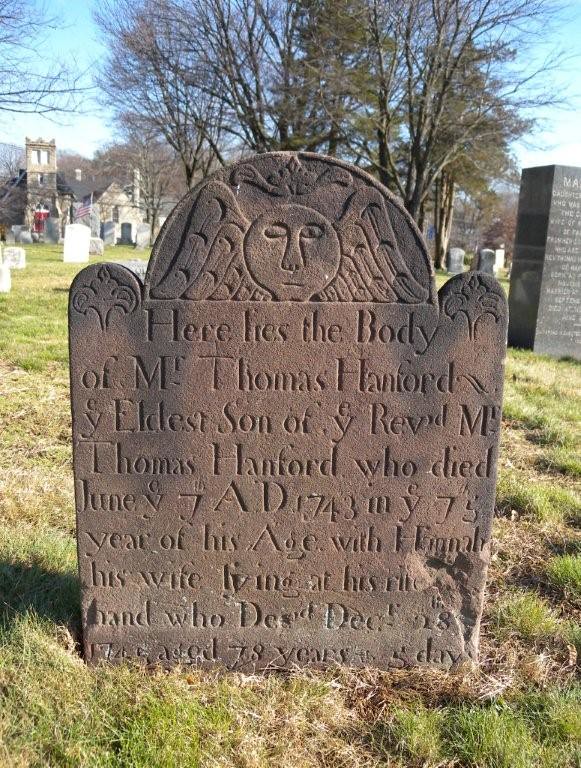This image captures a historic cemetery scene featuring a prominent headstone dedicated to Mr. Thomas Hanford, the eldest son of Reverend Thomas Hanford, who passed away on June 7th, 1743, at the age of 75. The headstone, constructed of a brownish-gray stone, stands tall and rectangular, crowned with a large semicircular top adorned with an engraving of a sun bearing a serene face with angel wings. The tombstone is placed in a grassy area, with patches of brown amidst the green, signaling the passage of time.

Behind the headstone, several tall trees—with some barren and others lush with pine needles—stand against a bright blue sky. The cemetery is dotted with other tombstones, and in the distance, there is a church building characterized by a tower with a cross. The church's architecture is intricate, with light brown and gray hues that blend into the bucolic setting. An American flag accompanies Mr. Thomas Hanford’s headstone, adding a touch of solemn patriotism to the serene and reflective atmosphere.